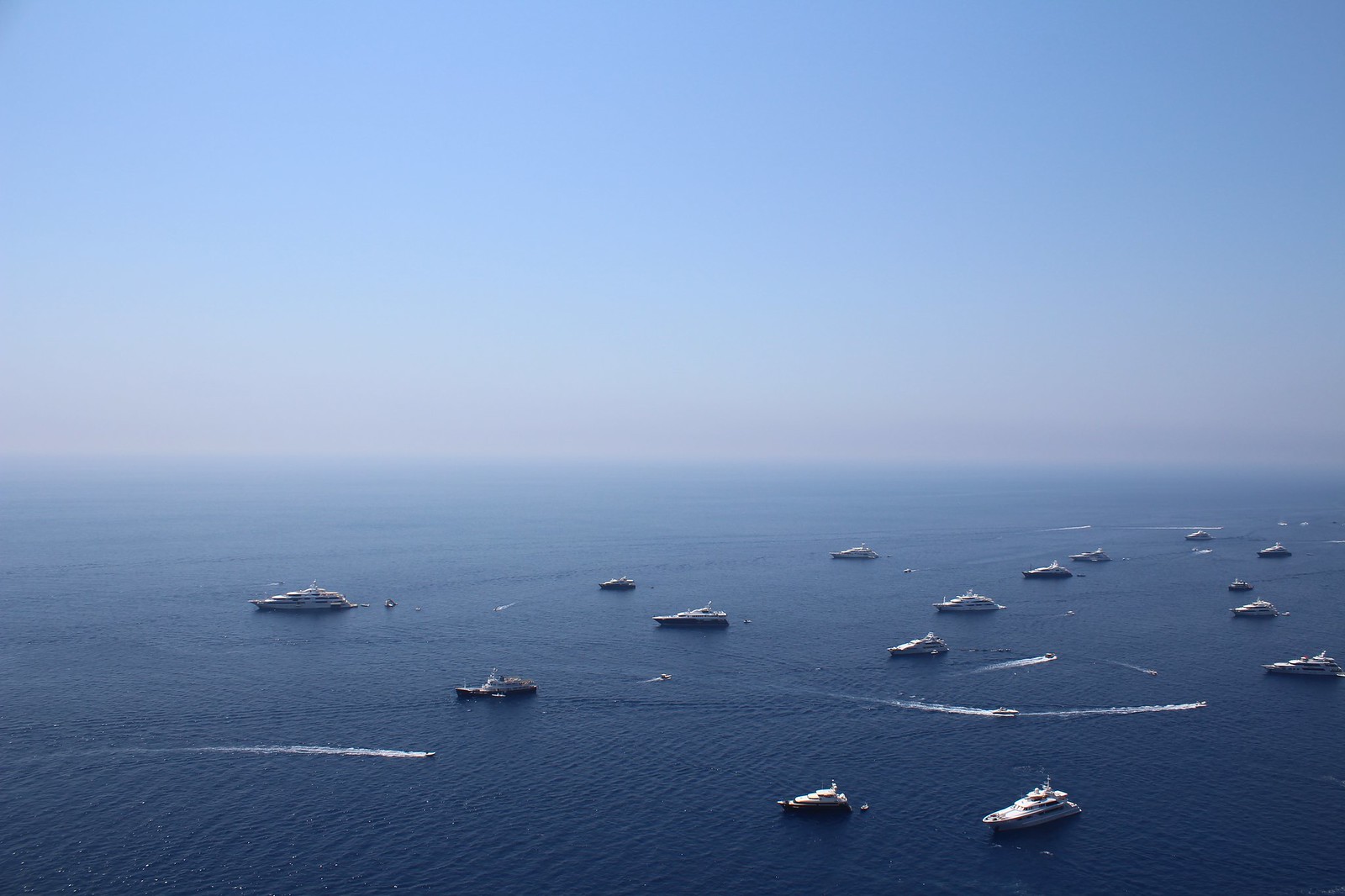This aerial photograph captures a stunning view of a group of yachts anchored in the middle of the deep blue ocean, likely taken from a great height such as a helicopter or cliff top. The image is bathed in a gradient of blue, transitioning from a darker shade in the bottom right corner to a lighter hue where the sea meets the misty, foggy horizon. The sky above is a clear blue, contrasting beautifully with the expansive sea below. Scattered across the ocean are numerous large yachts, arranged in a staggered pattern, along with speed boats and perhaps some patrol boats navigating around them. Visible amongst the yachts are jet skis, leaving white water trails as they zip around, suggesting a dynamic activity, possibly a race. The luxury of the yachts and the overall composition exude an atmosphere of opulence and grandeur amidst the vast, open sea.